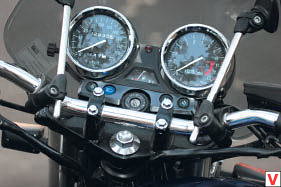This image showcases a close-up view of a motorcycle control panel against a grey background. Dominating the scene are two large, circular dials with chromium surrounds, which bring a touch of vintage elegance to the panel. One of these clearly functions as a speedometer, its hands prominently displayed, while the purpose of the second dial remains less clear. The handlebars, made of polished chromium, provide a striking contrast and add to the overall aesthetic appeal. 

Nestled between and beneath these primary dials is a backboard featuring an array of smaller gauges and indicators, each clamped securely in place. Below the central handlebars, a substantial chromium knob is prominently visible, accompanied by a black plastic attachment whose function is not immediately apparent. Flanking the sides of the dials are two upright metallic bars, whose precise roles remain obscure, adding an element of intrigue for viewers unfamiliar with motorcycle mechanics.